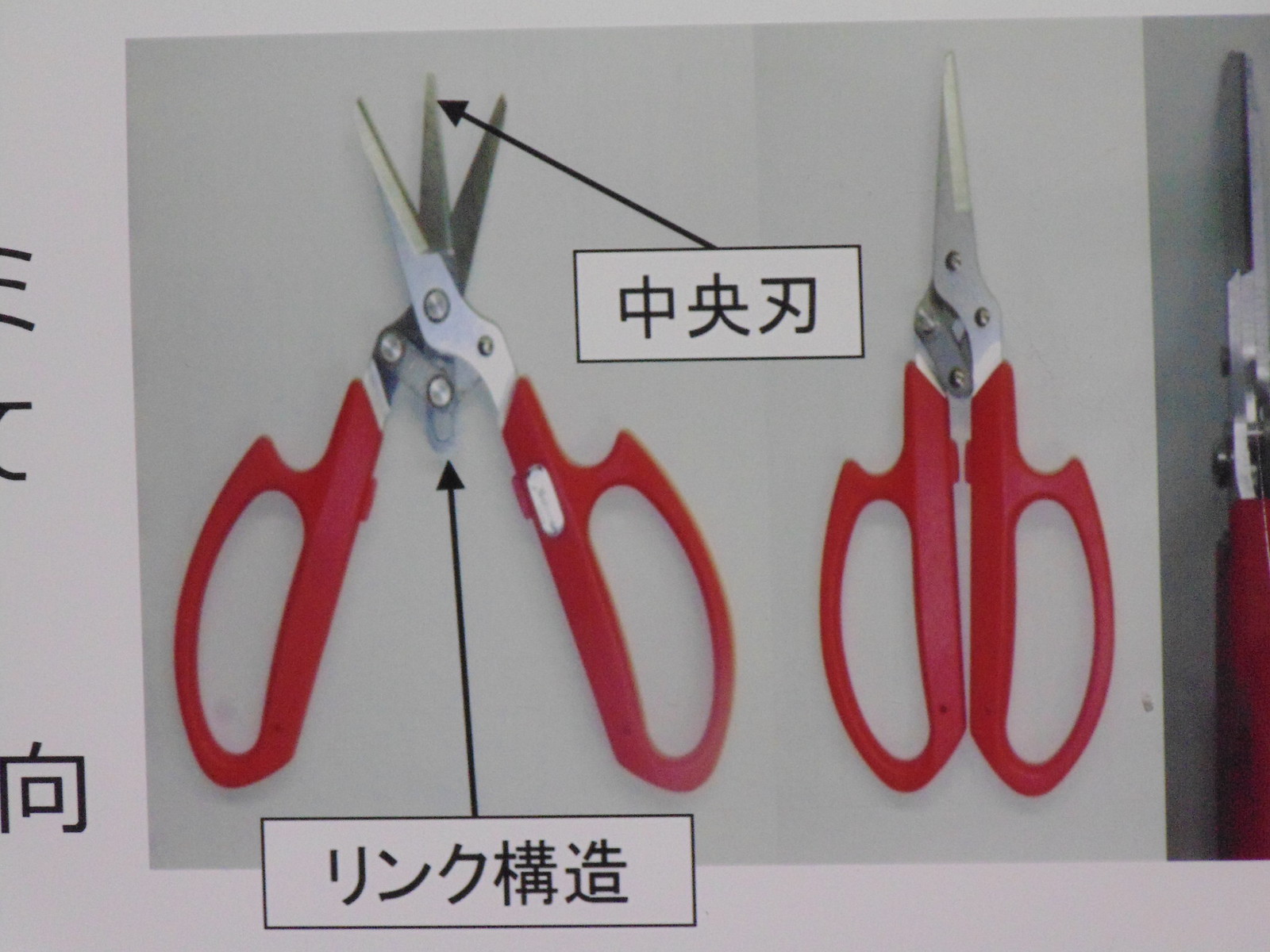The image displays two pairs of red-handled scissors with gray steel blades against a light gray background, positioned centrally within a white-bordered rectangle. The left pair of scissors is open, while the right pair is closed. Superimposed are two rectangular boxes featuring foreign text, possibly Chinese or Japanese, both pointing towards the open scissors on the left. Above the left side of these text boxes, there's a logo consisting of a smaller square inside a larger square and some black lines that appear cut out. In the bottom right corner, part of a red object is visible, partially covered by the gray background.